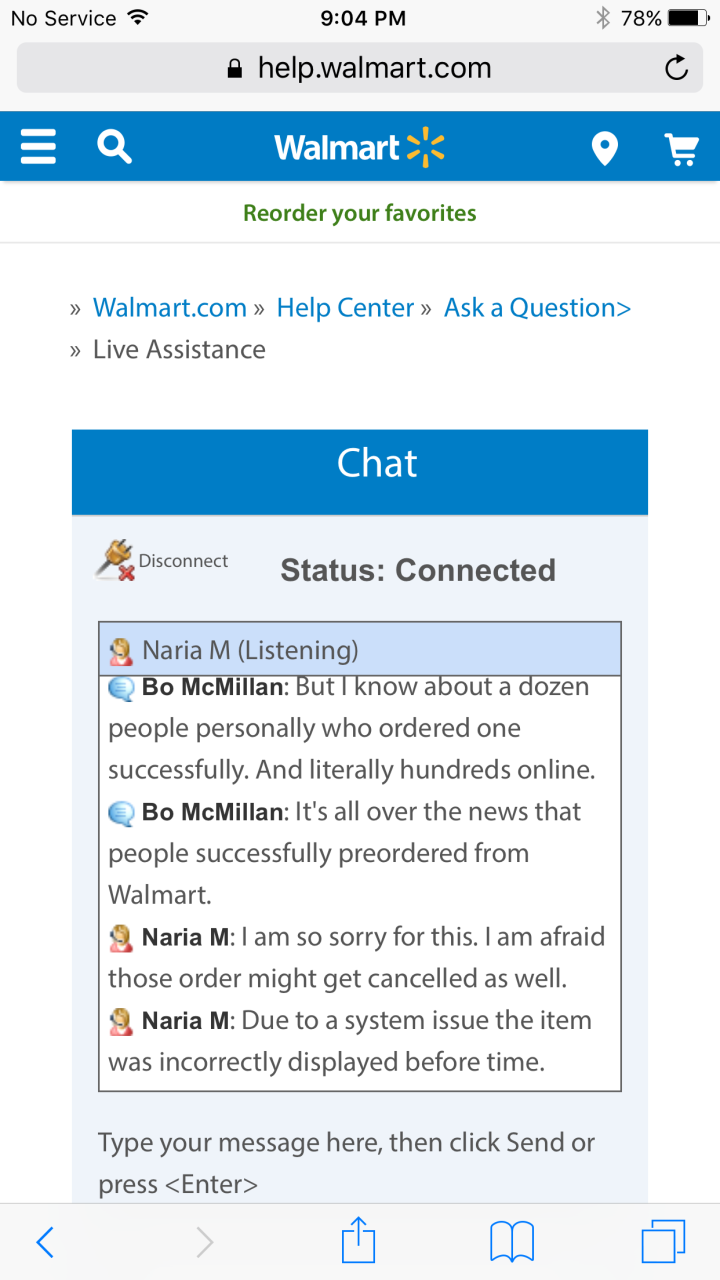The image depicts a chat screen on a smartphone, specifically a customer service chat with Walmart. At the very top of the screen, there is a gray bar displaying the URL "help.walmart.com". Below this, a blue bar features the Walmart logo on the left in white letters, with the yellow flower-like emblem to the right. To the right of the logo, there are several icons: a shopping cart, a location pin, and a search bar. On the left of the logo, there is a search icon and three horizontal white bars indicating a menu.

Beneath this blue bar, the rest of the screen has a white background. Immediately below the Walmart logo, a green text reads "Reorder your favorites." Following this, in blue text, there are the links "walmart.com help center" and "ask a question." Further down, in black text, it says "live assistance." 

A thick blue bar below these texts states "chat" in white letters. Under this bar is the chat log between two individuals, Bo McMillan and Naria M. Bo McMillan's comments are displayed first, followed by responses from Naria M. The chat log contains multiple lines of text, showing an ongoing conversation between the two.